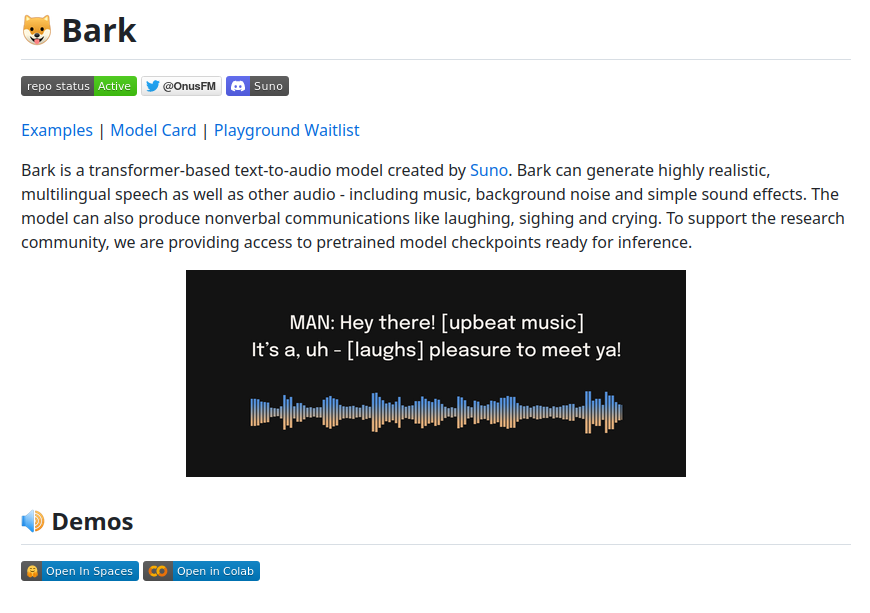The image is a screen capture from a website with black text on a white background. At the top left, there's an emoji of a dog, which appears to be either a Shiba Inu or a Corgi, depicted as a brown dog with white markings around its face. Adjacent to the emoji is the word "bark" in black text.

Below this, several icons are displayed: "Repo status: active," a Twitter symbol with the handle "@OnusFM," and a Discord symbol followed by "Suno." 

Further down, there are links formatted in blue text: "Examples," "Model card," and "Playground wait list." 

Underneath these links, a paragraph in black text explains:

"Bark is a transformer-based text-to-audio model created by Suno (with 'Suno' in blue). Bark can generate highly realistic multilingual speech, as well as other audio, including music, background noise, and simple sound effects. The model can also produce nonverbal communications like laughing, sighing, and crying. To support the research community, we are providing access to pre-trained model checkpoints ready for inference."

At the bottom of the image, there is a black rectangle featuring white text and a sound bar. The text reads: "Man: 'Hey there,' [upbeat music] 'It's a, uh,' [laughs] 'pleasure to meet ya.'"